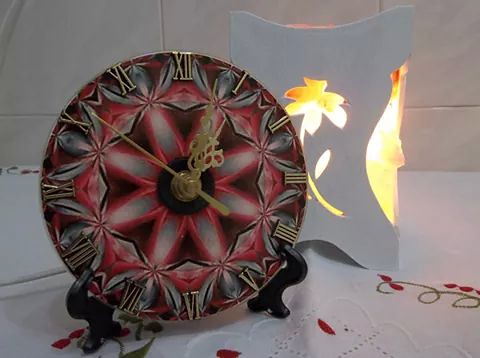The photograph features an ornate analog clock set against a white tile background. The clock, which stands on dark black legs, has a face characterized by a red and grey starburst pattern. The Roman numerals marking the hours are crafted in a brassy gold color and the hands, also brassy gold, have intricate, fancy designs. At the center of the clock is a red shape resembling a starfish, bordered in red and filled with grey. To the right of the clock is an off-white, rectangular lamp with gently curved edges. This lamp has a cutout design of a flower and stem, through which a warm yellow-orange light shines. The scene is set on a white floor scattered with a white napkin adorned with tiny red dots and a green swirl.